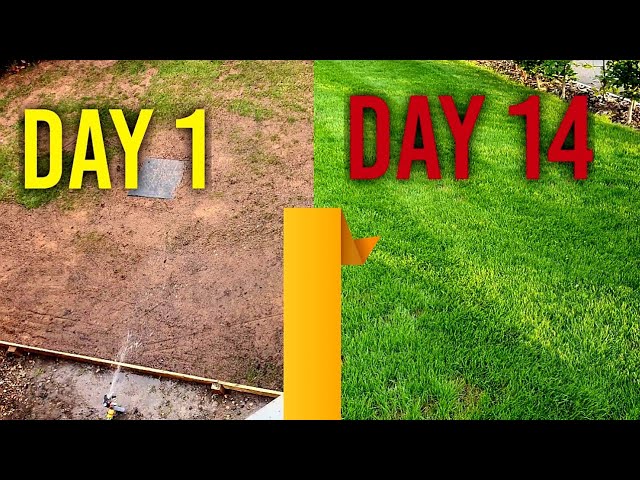The image is a side-by-side comparison of a lawn transformation, vividly illustrating a two-week period of improvement. The left-hand side, labeled "Day 1" in bold yellow text, shows a barren landscape predominantly composed of dirt with very sparse patches of grass. A sprinkler head can be seen watering this sparse area, and there is some wood at the bottom, possibly part of a raised garden bed. The right-hand side, labeled "Day 14" in bold red text, reveals a dramatic transformation into a beautiful, lush green lawn with no bald spots. The grass appears freshly mowed, and in the upper right corner, there is a glimpse of brown beauty bark or mulch with small plants or shrubs growing, adding to the rich, verdant appearance. The two images are partially separated by a yellow ribbon-like strip, enhancing the visual contrast between them. The entire photograph is framed with solid black bars at the top and bottom, giving it the appearance of being presented on a widescreen display.